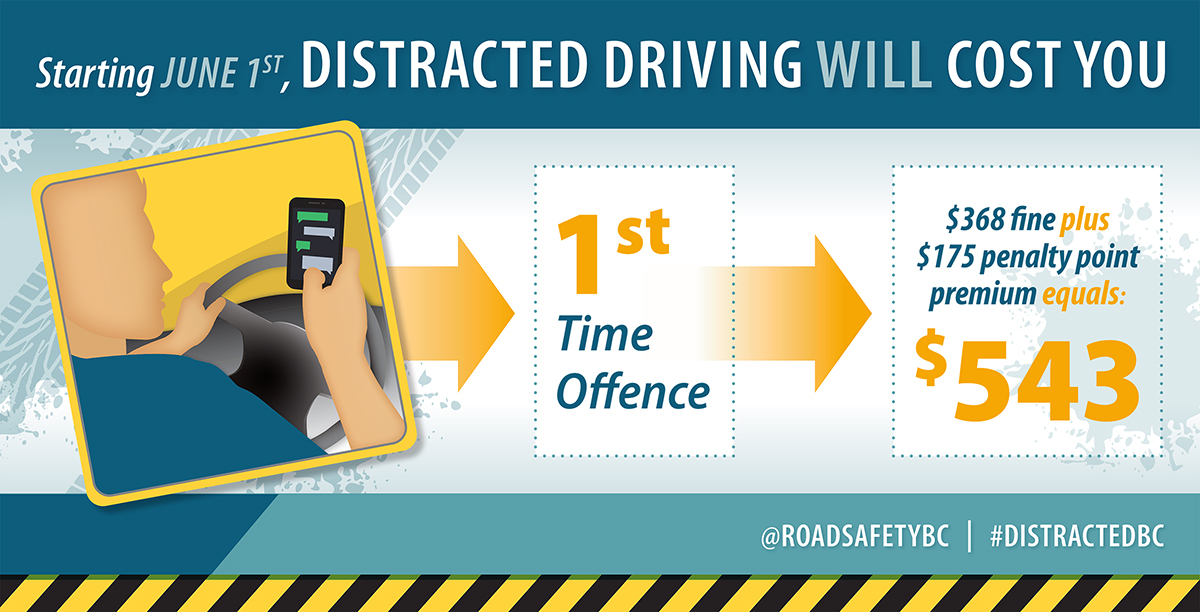This is a road safety public service announcement about the dangers and penalties of distracted driving. The graphic likely shared on social media, flyers, or television, prominently features a teal-colored banner at the top with the text, "Starting June 1st, distracted driving will cost you." The main illustration is a simple cartoon of a man driving with one hand on the steering wheel and the other on his phone, depicting him texting. An arrow points to a text block reading "First-time offense," followed by another arrow detailing the fines: a $368 fine plus a $175 penalty point premium, totaling $543. At the bottom, a teal banner displays "Road Safety BC" and the hashtag "distracted BC," underlined by a hazard bar with yellow and black stripes for emphasis.